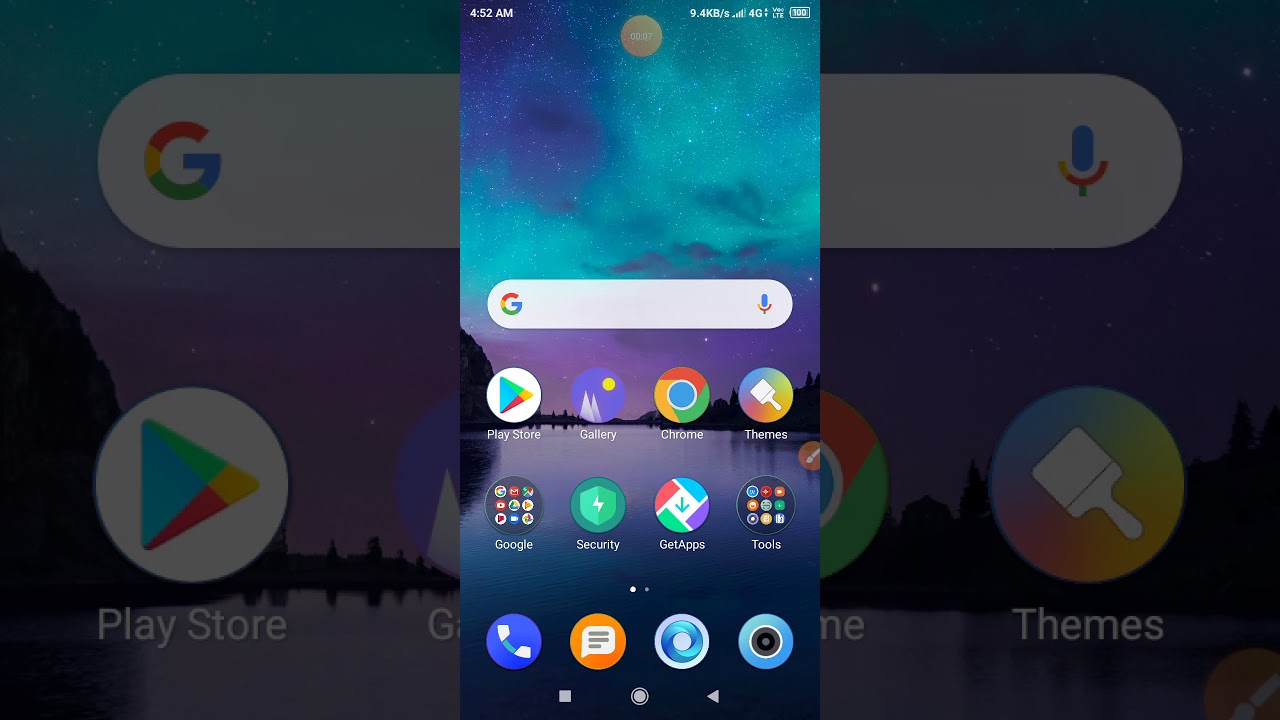The image showcases a digital device screen, likely a smartphone or tablet, with a slightly faded appearance. At the top of the screen, there is an empty Google search bar. Below the search bar, a grid of 12 app icons is arranged, with a layout of four apps per row and three rows in total. The background of the screen features a standard blue hue with a faint landscape image.

Interestingly, superimposed in the center of this screen is a duplicate image displaying the same screen layout. This overlay is highly exposed and significantly zoomed in, showing only the top row of the app icons. Despite the exposure, it's clear that the duplicate image maintains the same structural elements as the primary screen, including an identical Google search bar at the top and a matching blue landscape background.